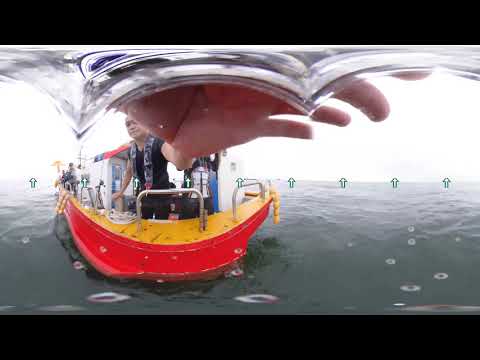The image depicts an individual on a boat, possibly a tugboat, floating in a calm ocean or lake. The boat features red sides and a yellow deck, equipped with handrails encircling it. The primary figure, an Asian man wearing a black shirt and pants, is standing at the bow, reaching out and seemingly holding a camera, possibly taking a selfie. The boat’s deck is cluttered with various tools, wires, and other equipment, hinting at some form of work or maintenance activity. There are additional people visible in the background, engaged in their own tasks. The scene is enveloped in an overcast or foggy atmosphere, with a white sky obscuring the horizon. Digital green arrows pointing upwards overlay the horizon, adding a curious element to the image.